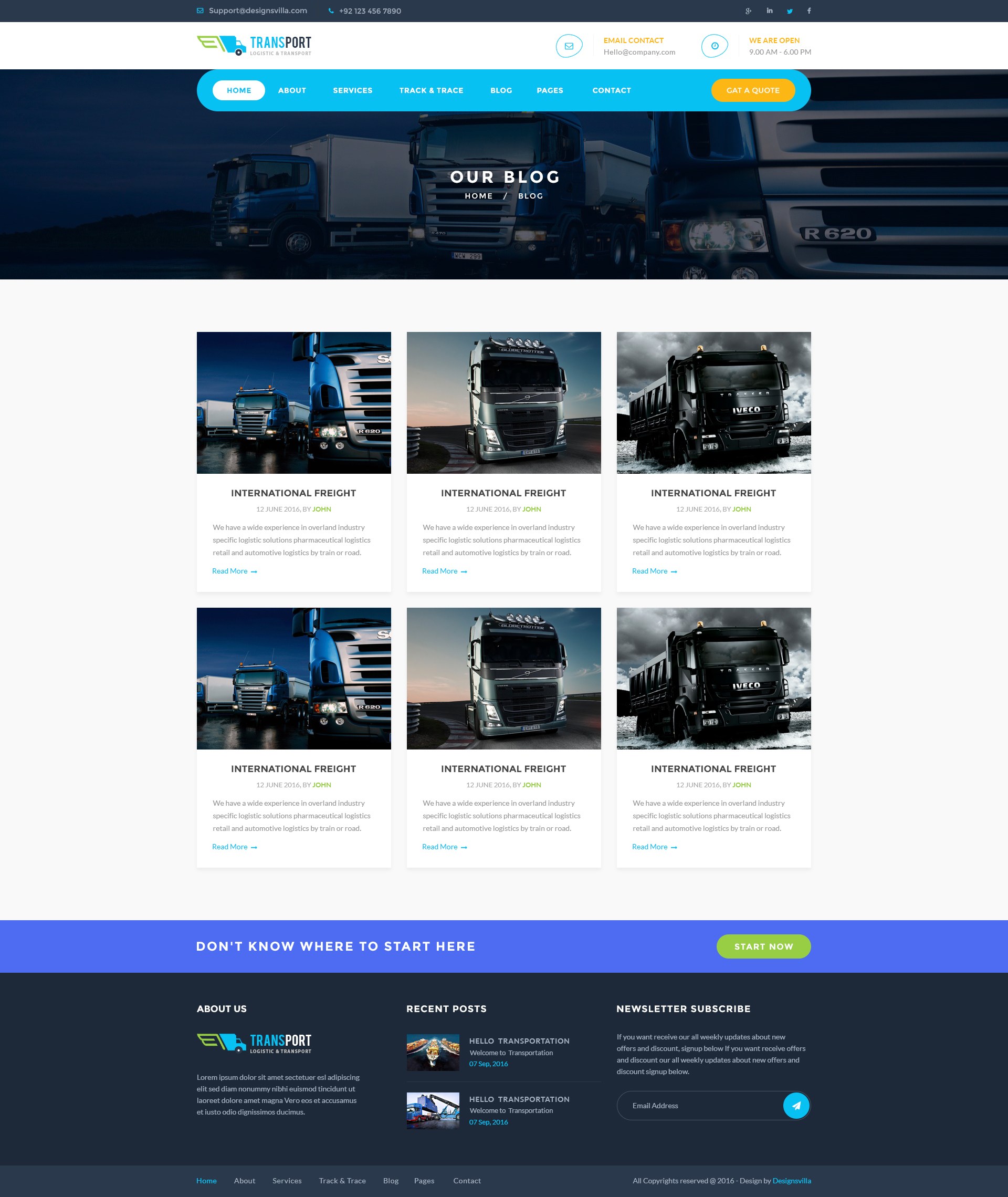The image features a blue gradient background at the top transitioning to white. At the top, in white text, is the email address "support@designvilla.com" followed by the phone number "+921-234-567-890." Below this, there are icons for social media platforms including Google Plus, LinkedIn, Twitter, and Facebook.

The background changes to white where a blue truck with a green rear section is prominently displayed. Beside the truck, the word "Trans" is written in blue and "Port" in black, suggesting the name 'Transport' for the business. Underneath, in smaller text, it appears to read "Logistics" and "Transport."

On the right side, in yellow text, the email contact information is displayed as "hello@company.com." Below this, in orange text, it says "We are open," followed by "9:00 AM to 6:00 PM" in black text.

A blue oval contains various navigation tabs. A highlighted white oval around the "Home" tab indicates the active page. Other tabs include "About," "Services," "Track and Trace," "Blog," "Pages," and "Contacted," the latter highlighted in an orange oval labeled "Get a Quote" in white text.

Beneath this, an image of three lined-up trucks is overlaid with the text "Our Blog Home / Blog" in white. The page appears to be devoted to international freight, showcasing two rows of three blog posts each.